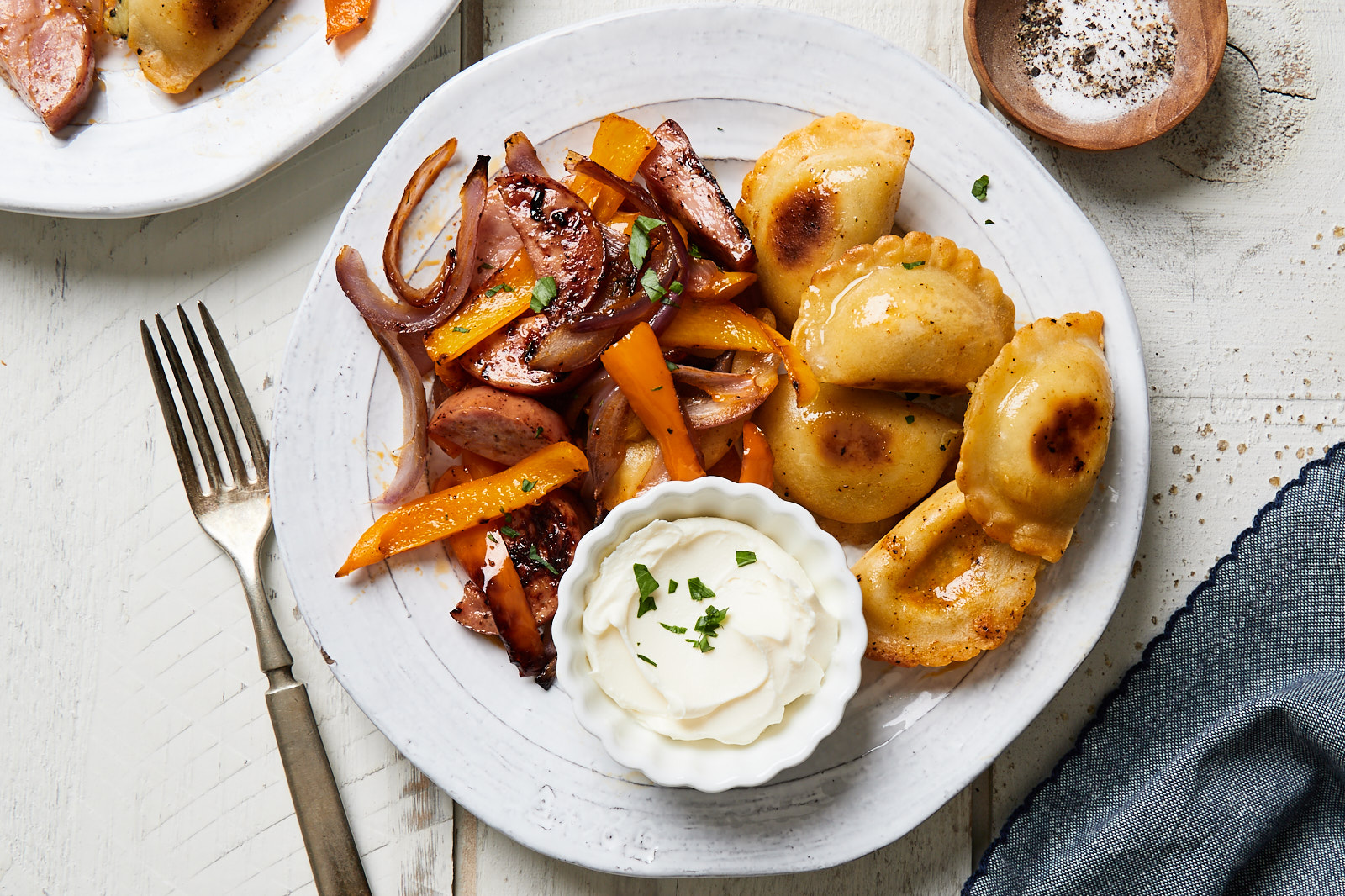This is a detailed color photograph in landscape orientation, captured from a top-down perspective. At the center of the image sits a round white plate adorned with various foods. On the right side of the plate, there are five hand-rolled pierogies, each featuring a dark brown indentation on top and a scalloped edge. To the left, there is a selection of roasted vegetables, including carrots, onions, and potatoes. At the bottom of the plate, a white souffle cup filled with a creamy substance, likely sour cream, garnished with green chives, completes the dish's presentation.

Adjacent to the plate on the left side is a silver fork, angled with its handle pointing downward towards the bottom of the image. In the upper left corner, the edge of another white plate is partially visible. To the top right of the main plate, a small brown wooden bowl, possibly containing additional white sauce, rests on the table. The background is a white table adorned with a white lacy fabric peeking out in the lower right corner. The photograph showcases a realistic and detailed representation of the food, following the style of photographic representationalism and food photography.